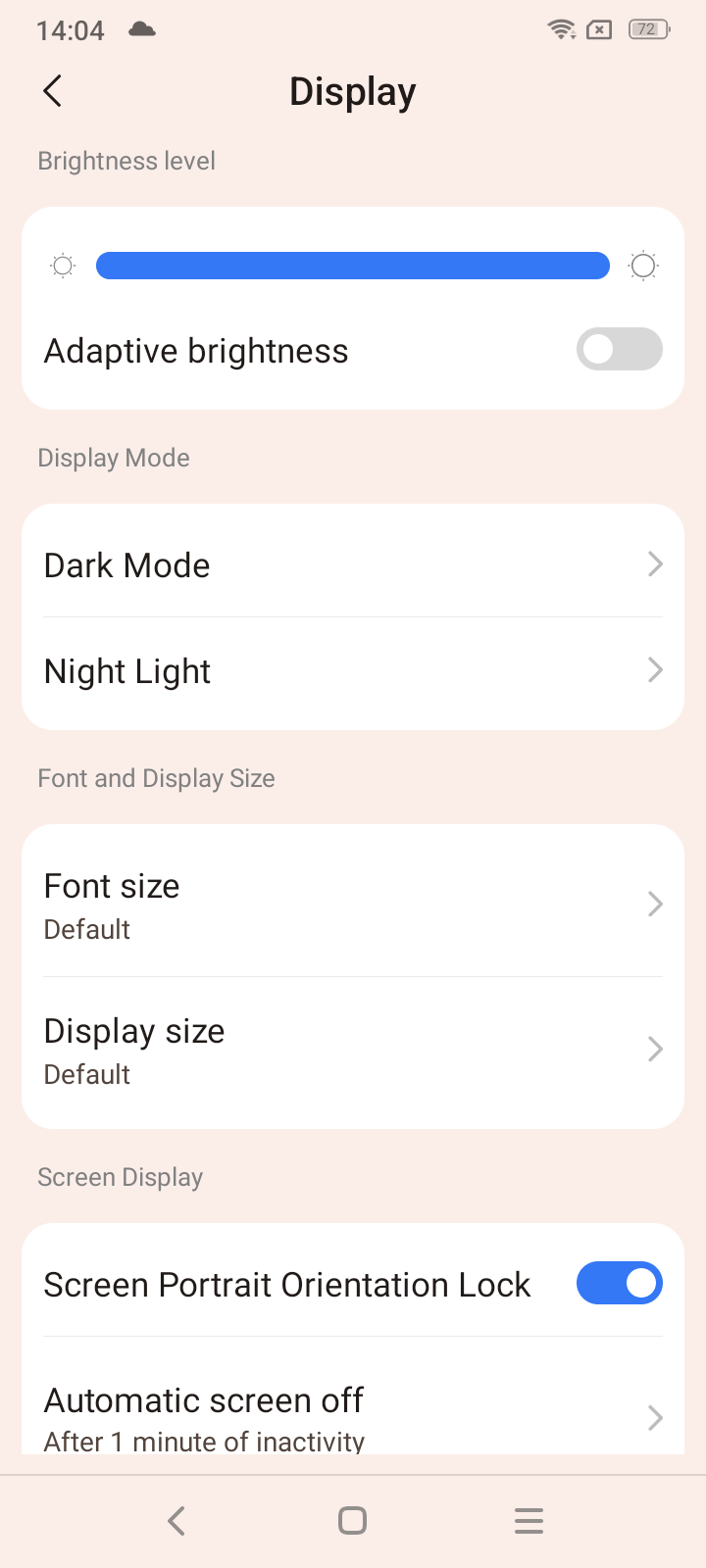This image appears to be a screenshot of a smartphone's display settings captured on a device with a pink background. In the status bar at the top left, the time reads "14:04," accompanied by a Wi-Fi signal icon and a partially filled battery icon on the right.

Below the status bar, there's a navigation arrow pointing left with the word "Display" adjacent to it, indicating the current settings category.

The first section titled "Brightness level" contains a white rectangle with a blue adjustment bar across it. Beneath this, "Adaptive brightness" is displayed with an on/off toggle switch, which is currently turned off.

Next is the "Display mode" section. A white rectangular box presents two options: "Dark mode" and "Night light."

Following this, the heading "Font and display size" appears. A white rectangle offers two settings: "Font size: Default" and "Display size: Default."

The subsequent heading, "Screen display," includes a white rectangle labeled "Screen portrait orientation lock" accompanied by a toggle switch, which is toggled on. Additionally, the setting "Automatic screen off after one minute of inactivity" is mentioned below it.

At the very bottom of the screen, there are navigation icons: an arrow pointing left, a square, and three vertical lines stacked on top of each other. These likely represent the phone's navigation buttons.

This screenshot meticulously details the options within the display settings, allowing users to customize their viewing experience on their device.